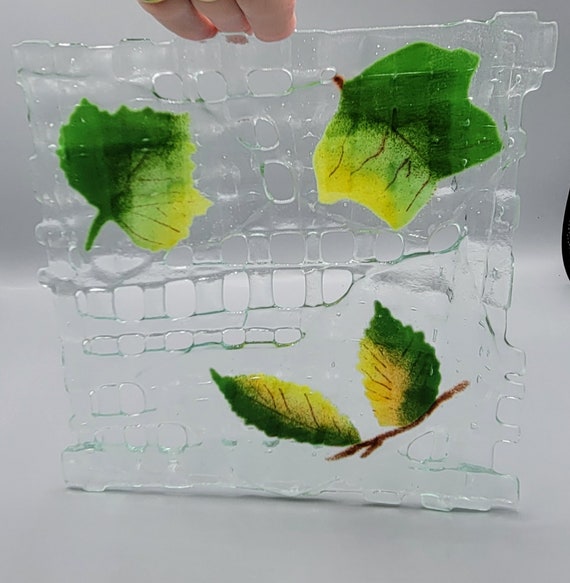This photograph captures a square, translucent object that is held up by three fingers at the top edge. The object, which appears to be either ice or plastic with a jagged border, encases three different types of leaves, preserving them in a delicate display. In the upper left-hand corner lies a leaf with a dark green hue on the left side transitioning into a lighter green on the right. Mirroring this, the upper right-hand corner houses a similarly patterned leaf with dark green on the right half and lighter green to yellowish tones on the left. At the bottom right, a small brown stem holds two smaller leaves that also exhibit a gradient from dark green to light green and yellow, each detailed with prominent brown veins. The translucent medium around the leaves features scattered holes, adding to the textured appearance of the display. The photograph, devoid of any text or words, is likely taken indoors, showcasing the preserved leaves in a straightforward, front-facing view.